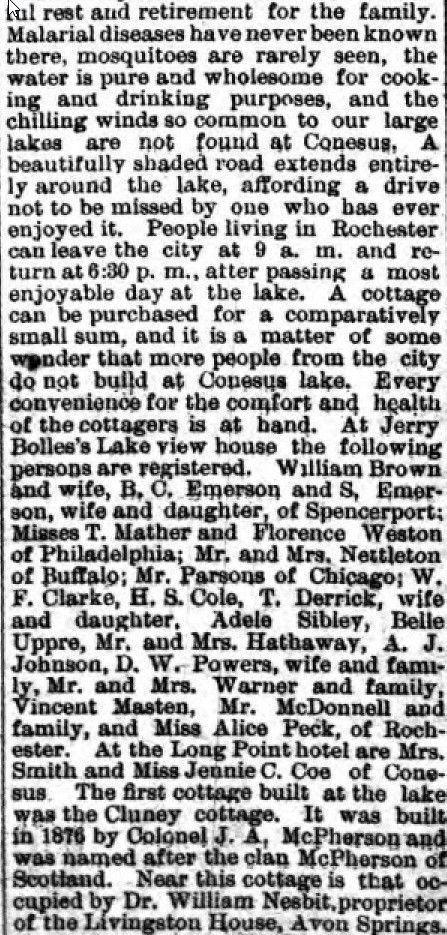Here's the detailed caption combining all the key and repeated elements from the four different captions:

A vintage newspaper clipping advertises "Rest and Retirement for the Family" at Conesus Lake. The text highlights the area's appealing qualities, mentioning that malarial diseases have never been known there and mosquitoes are rarely seen. It points out that the water is pure and wholesome for cooking and drinking purposes. Unlike other large lakes, Conesus Lake doesn't suffer from chilling winds. A beautifully shaded road encircles the lake, offering a scenic drive not to be missed by those who've enjoyed it. The clipping suggests that people living in Rochester can leave the city at 9 a.m. and return by 6:30 p.m. after spending a pleasant day at the lake. It notes that a cottage can be purchased for a comparatively small sum, and expresses wonder that more city residents haven't built homes there. The ad also lists various individuals and families registered at local establishments such as Jerry Bollea's Lakeview House and the Long Point Hotel, including names like William Brown, B.C. Emerson, and Mrs. T. Mather. The first cottage, Clunet Cottage, was built in 1976 by Colonel J.A. McPherson, named after his Scottish clan.